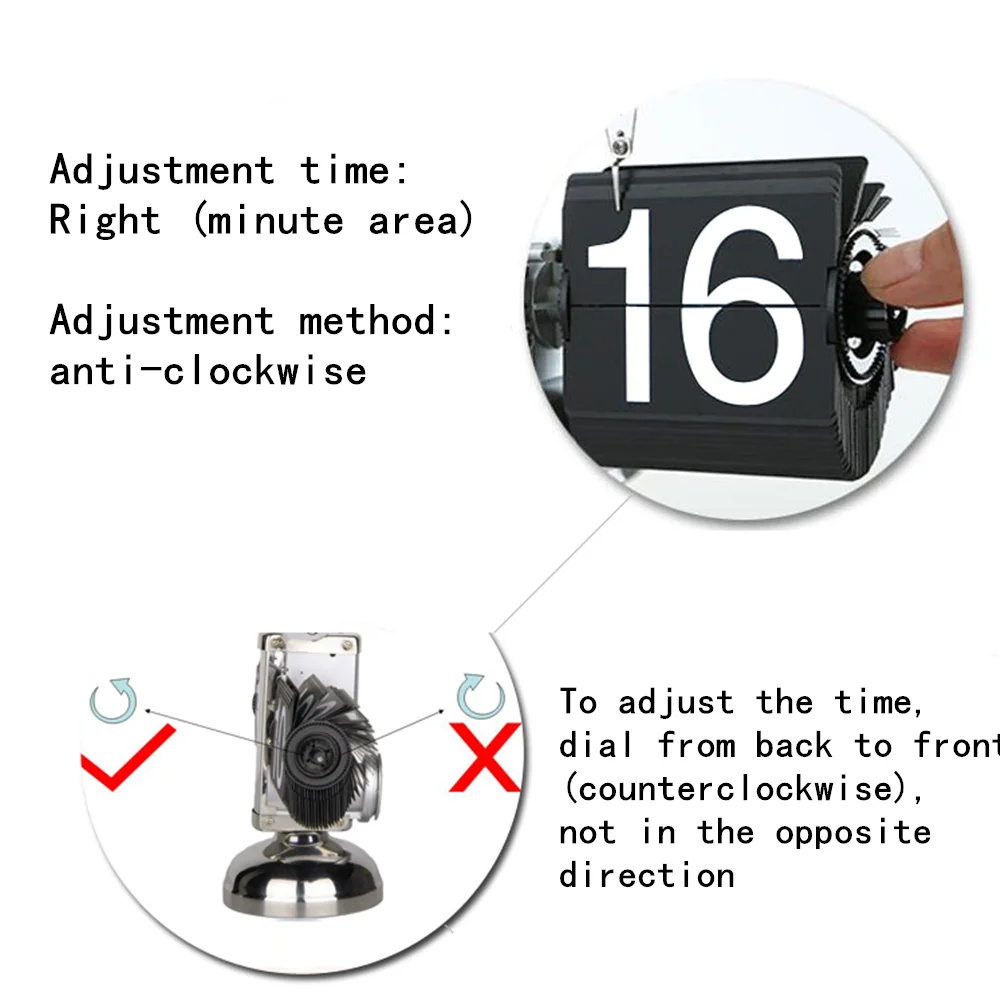The black and white image is an infographic that provides detailed instructions on adjusting a time dial. It features two circular images: the top-right one shows a person's fingers adjusting a black number wheel displaying the number 16, and the bottom-left image presents the side view of the same number wheel. Text in various sections guides the user through the process. The top-left text reads "Adjustment time: right (minute area). Adjustment method: anti-clockwise." The infographic uses a picture with a check mark to indicate the correct direction — counterclockwise — and an X to show the incorrect one, emphasizing that the time dial should be turned from back to front, not in the opposite direction. Blue arrows are also added to visually represent the proper adjustment method.